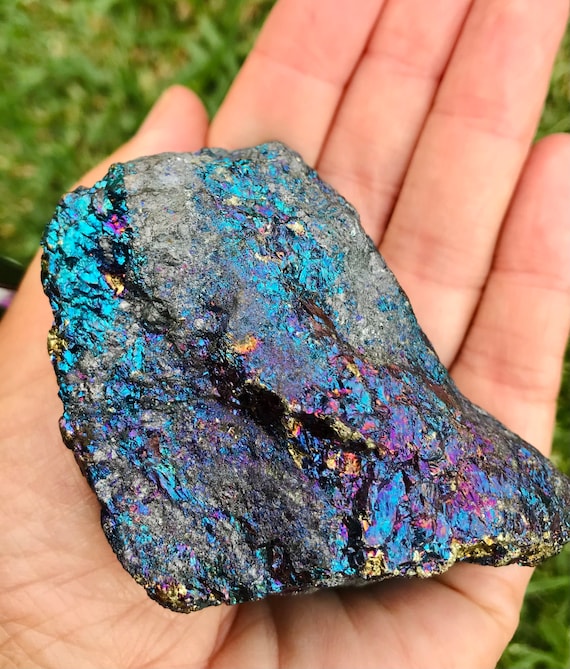This image is a close-up photograph of a unique, dark-colored rock held in the open palm of a light-skinned person's left hand. The hand, oriented slightly upward to the right, dominates the frame, with fingertips extending out of the image. The thumb is visible on the left side, guiding the curved shape of the rock, which spans from just beneath the thumb nail to the bottom of the pinky finger, covering the majority of the palm. The rock is characterized by its jagged, triangular shape, pointing to the right, reminiscent of a boot but with a bowed bottom edge. 

The rock's surface is predominantly charcoal gray but exhibits a stunning array of iridescent colors. Notably, there are bright blue fluorescent patches near the thumb knuckle, purplish hues towards the bottom right where the pinky meets the palm, and tinges of yellow and gold scattered across its rough texture. The background features a blurred view of green grass, indicating that the photo was taken outdoors in daylight, possibly where the rock was found. The intricate details and vibrant colors of the rock make it a striking focal point within the photograph.